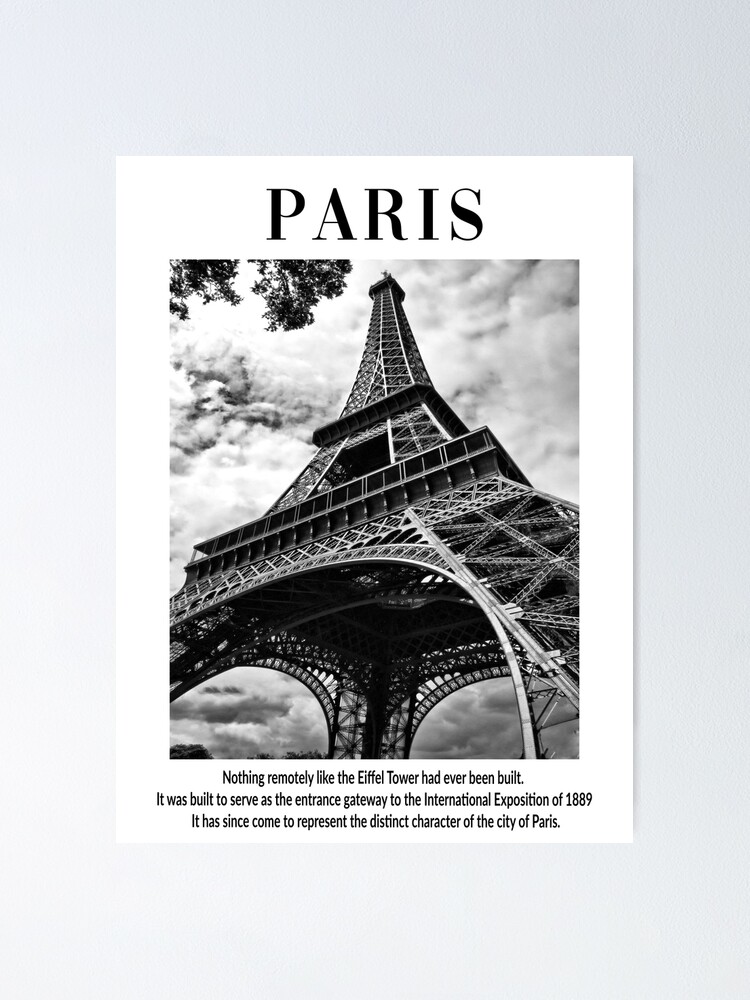A minimalist photograph displays a striking piece of wall art hanging against an off-white wall. The artwork features a pristine white canvas adorned with a black and white photograph of the iconic Eiffel Tower, captured from a unique vantage point directly beneath the structure, emphasizing its architectural grandeur as it ascends into a moody, cloudy sky. Above the photograph, bold black text elegantly reads "Paris," while directly below the image, smaller black text offers an insightful caption: "Nothing remotely like the Eiffel Tower had ever been built. It was built to serve as an entrance gateway to the International Exposition of 1889. It has since come to represent the distinct character of the city of Paris." The photograph subtly incorporates a hint of nature, with tree leaves peeking into the frame from the top left corner, adding depth and context.